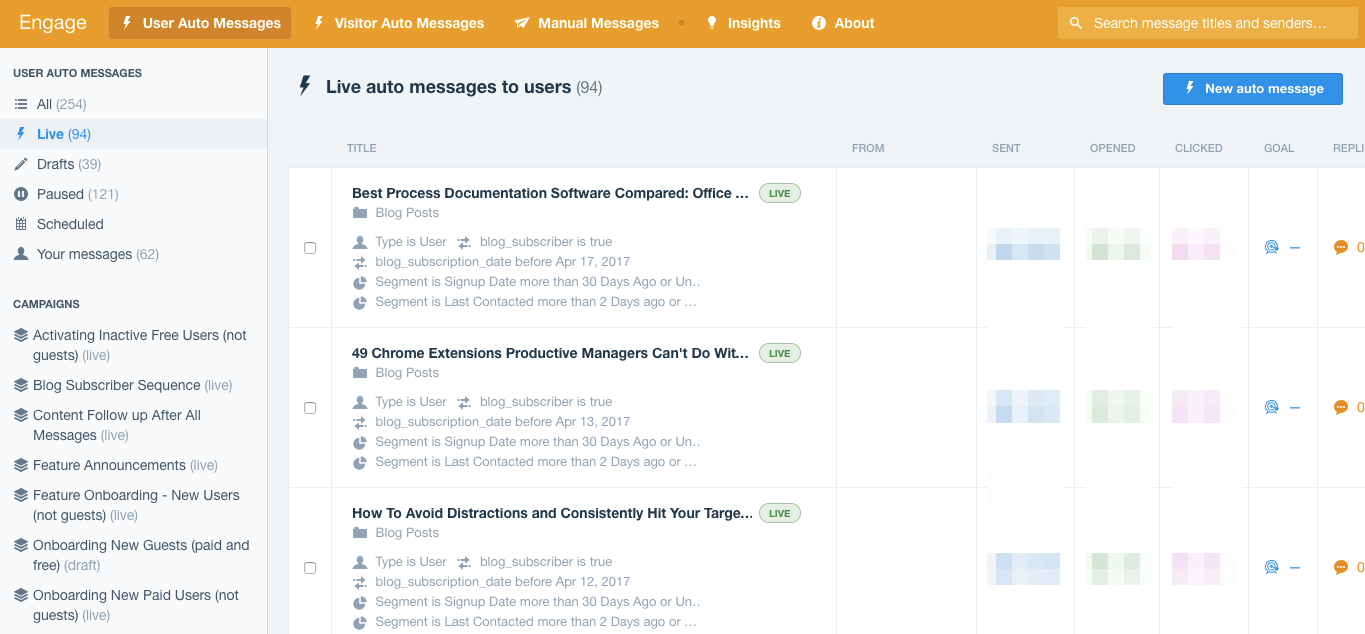The screenshot showcases a website interface, presumably named "Engage," which appears to be a messaging or automated response management platform. 

At the top, there is a prominent orange banner with white text. On the left side of this banner, "Engage" is displayed, potentially indicating the name of the website or webpage. Further to the right on the banner, several navigation buttons are visible, including "User Auto Messages," "Visitor Auto Messages," "Manual Settings," "Insights," and "About." At the far right end, there is a search box labeled "Search Messages, Titles, and Senders."

On the left side of the interface, there's a vertical toolbar or menu with options such as "All," "Live," "Draft," "Pause," "Schedule," and "Your Messages." Just below these menu items, there's a section titled “Campaigns,” listing various campaigns.

The main body of the webpage is dedicated to managing automated messages. At the top, it reads "Live Auto Messages to Users," with a blue "New Auto Message" button situated to the right.

Overall, this platform seems designed for creating and managing automated responses, likely for email or web-based communications.